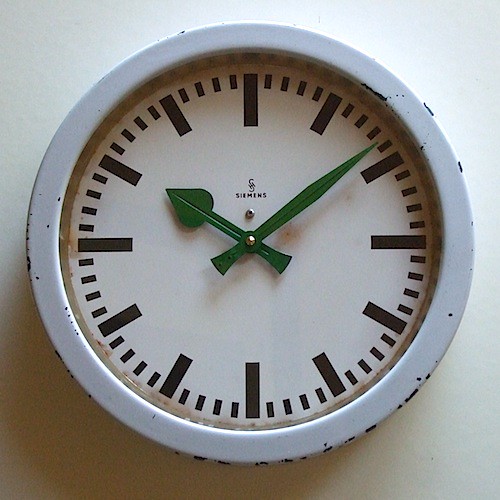This image captures a round wall clock mounted on a white background that transitions into a slightly darker shade towards the bottom, with the left corner of the image particularly darkened, likely due to shading. The clock is encased in a metal frame painted white, which has chipped significantly, revealing black areas beneath. The interior of the clock is also white, featuring large black bars to mark the hours and smaller black lines for the minutes, with no numerical digits. The clock's hands are green, with the minute hand being long and tapered, and the hour hand shaped like a spade. Positioned just below where the number 12 would be is the black text “Siemens,” printed above two silver screws that anchor the clock hands. The clock’s positioning casts a shadow down and to the left on the wall behind it, adding depth to the image.